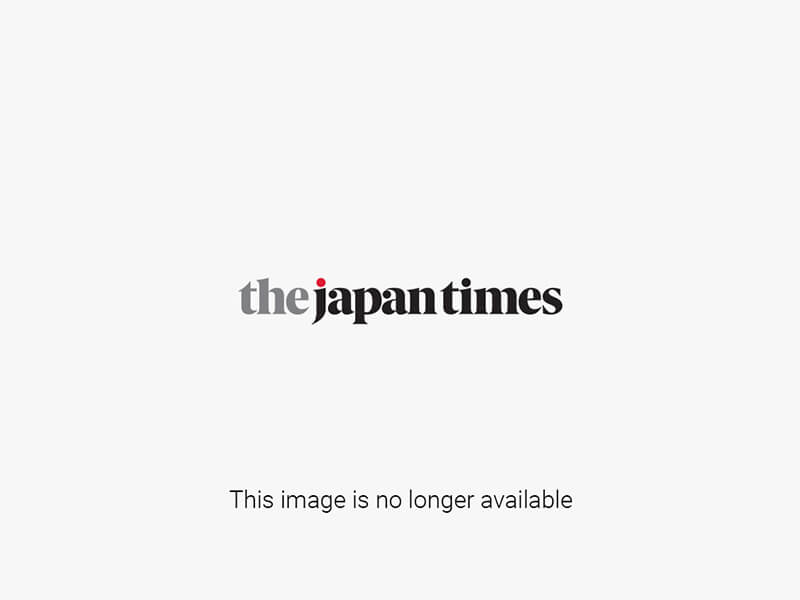This image captures a vibrant daytime ceremony taking place in Japan in front of a historic, two-tiered timber pagoda adorned with lights and surrounded by lush, green trees reminiscent of large bonsais. Spectators, though somewhat indistinct, line the sides, cheering and capturing the moment. The ceremony appears to be a parade, featuring rows of formally dressed individuals. The parade is led by men in white robes, followed by two men in intricate green robes carrying a large, beige crate-like structure that could be likened to the Ark of the Covenant. A notable figure in black attire follows, accompanied by another in a red robe. This ceremonial procession, set against the backdrop of traditional Japanese architecture and animated crowd, evokes a sense of cultural festivity and reverence.